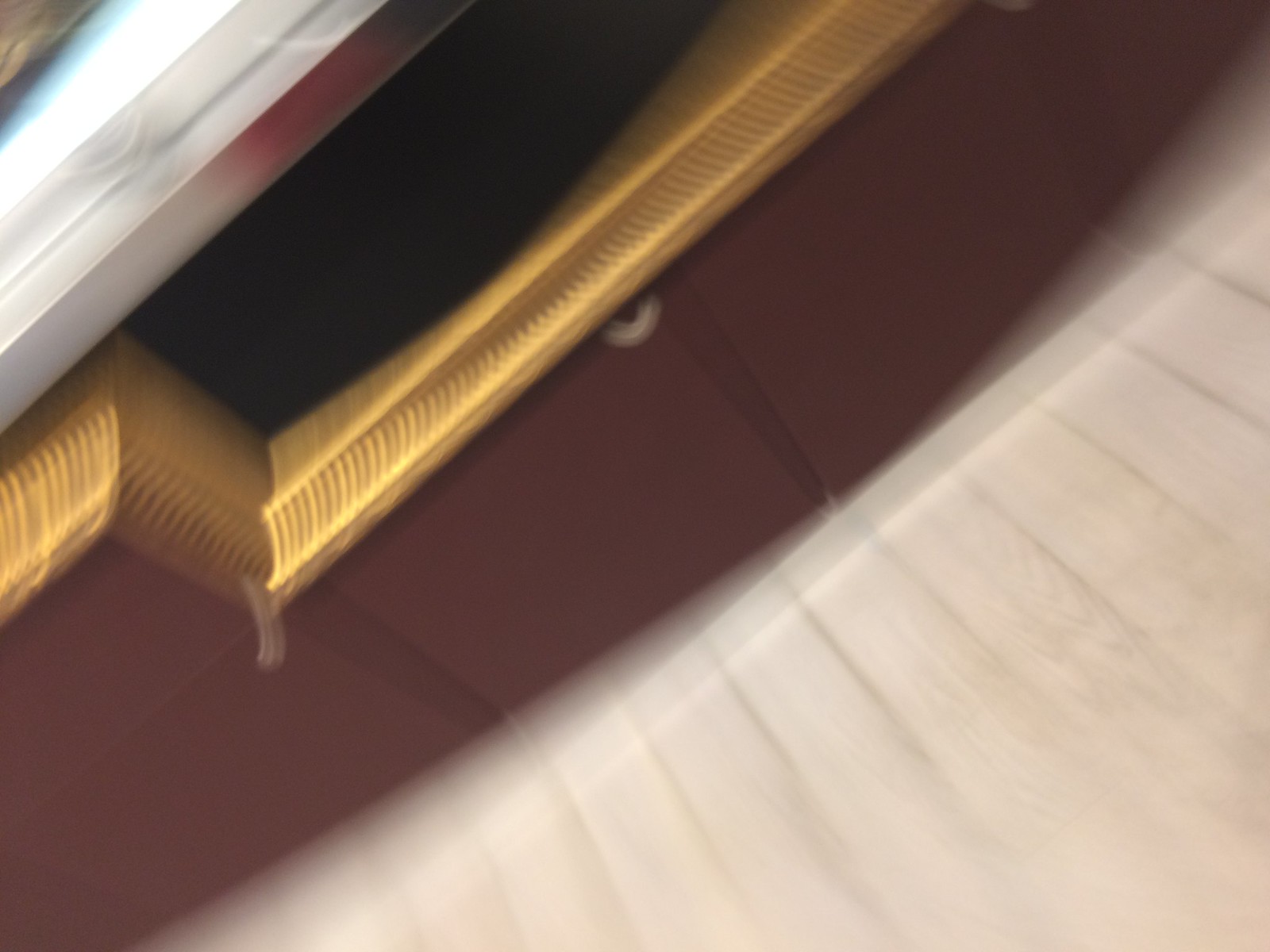The blurry image appears to show a kitchen or restaurant setting from a tilted side angle. The lower half of the picture features a pale, almost white, wooden floor. Above the floor, there are deep brown to maroon-colored cabinets that dominate the scene. These cabinets are adorned with a golden bamboo-like mat or layering. Additionally, a silver ledge or countertop is visible, possibly with a bright light attached to it. There's also an unidentifiable black object situated on or near the cabinets, adding to the complexity of the scene. The overall blur and motion effect make the details difficult to discern clearly.